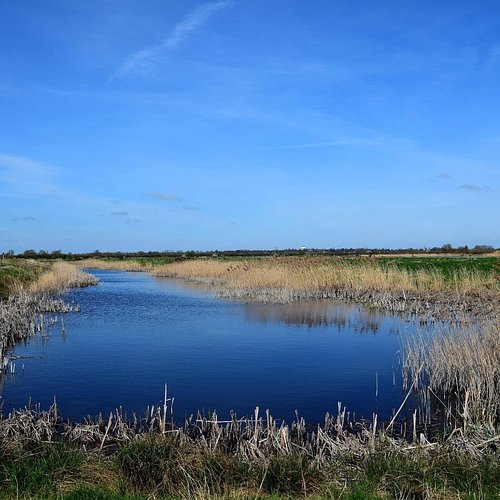A serene body of water is depicted in this image, possibly part of a slow-moving stream, as suggested by the reeds lining its banks and the marshy surroundings. The landscape appears to be a flat, delta-like plain with no significant peaks or valleys. In the distance to the far right, there are hints of minimal development, including a few structures, one of which is notably silver. The water itself is relatively still, with subtle movements detectable towards the left.